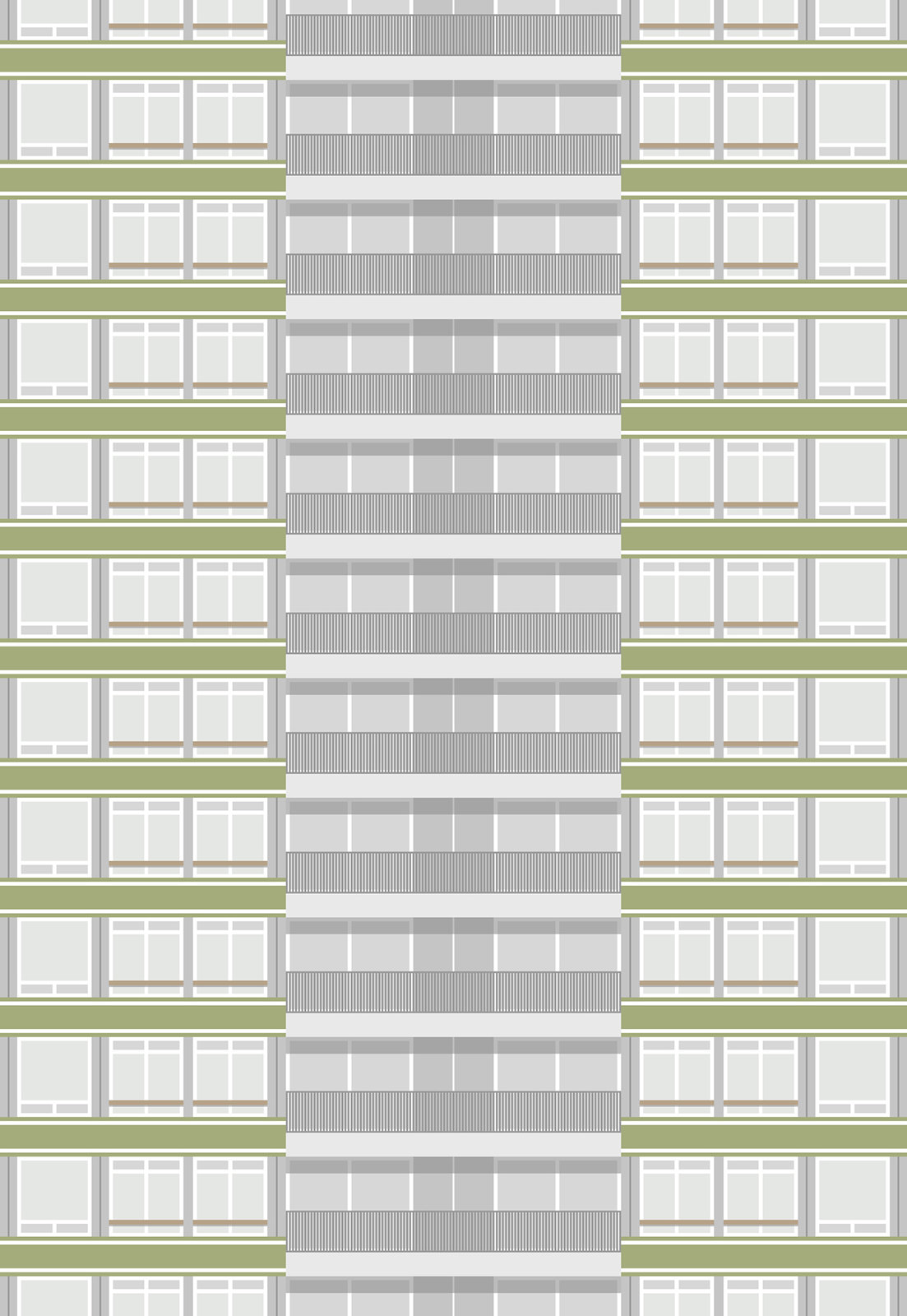This digital drawing illustrates the outside of a tall, vertical rectangular apartment building, captured in meticulous detail. The structure consists of about 10 to 12 stories. At the center of each floor, there is a sizable balcony with a black railing. Flanking these balconies, on either side, are three windows. The outer windows each feature one large pane with two smaller panes at the bottom. The inner windows, closest to the balcony, have a more complex design with four sections: two small panes at the top, two small panes at the bottom, and two rectangular panes in the middle. The central column of the building is highlighted in varying shades of gray, which contrasts with the olive green lines that demarcate each floor. This piece, with its simplified yet detailed design, serves as a graphic illustration likely intended for use on stock photo websites rather than a detailed architectural blueprint. The unified frame delivers an overall impression of a sleek, modern apartment building.